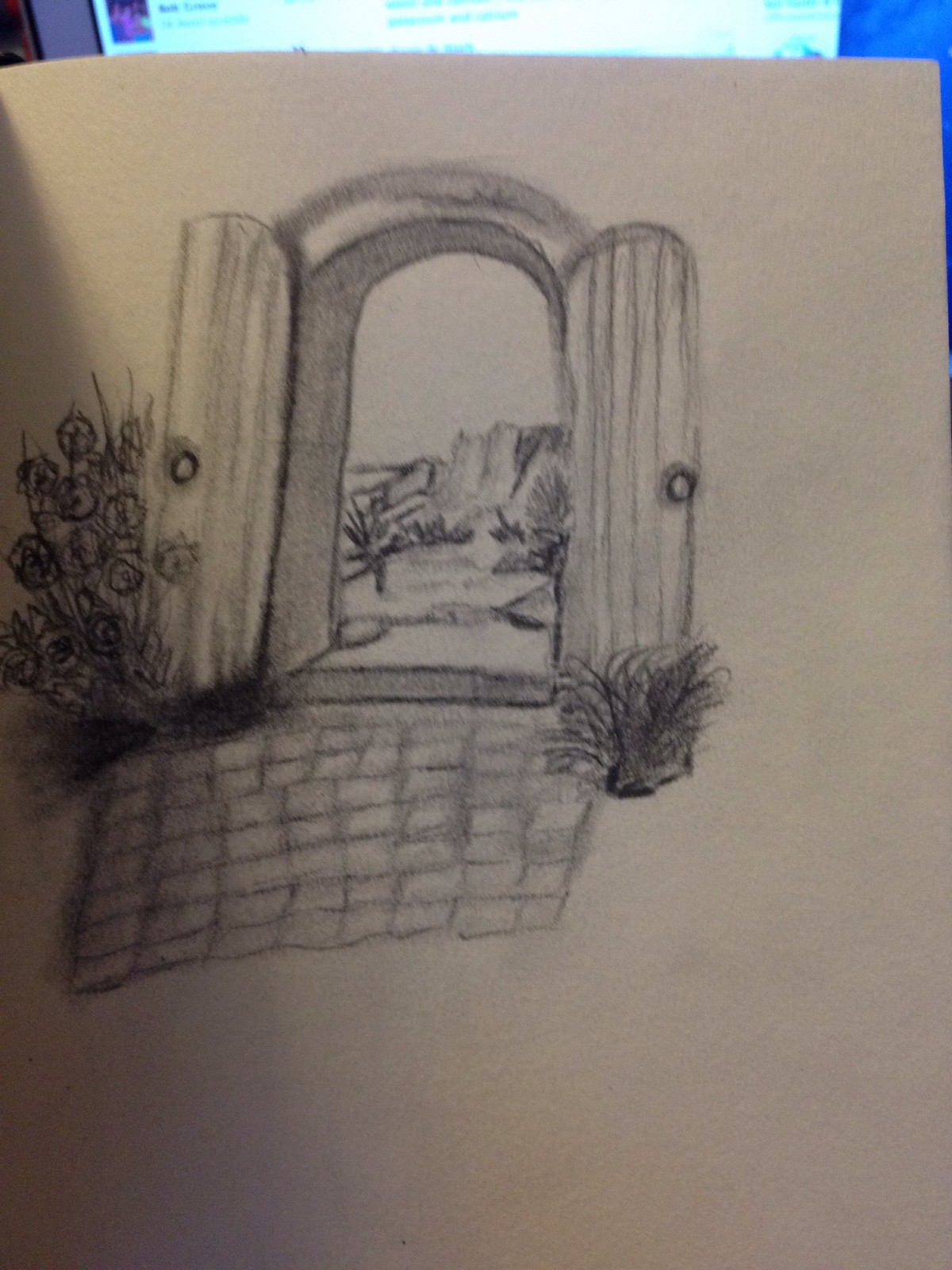The image is a detailed sketch, done on light brown, off-white sketchbook paper, likely with a charcoal or lead pencil. The focus is an arched doorway with two wooden, partially open doors, where the top of the doors are oval and the bottom squared off. The doorway features long lines indicative of wooden boards. Surrounding the archway, different shades of gray and hints of white are used to give depth. Leading up to the doorway is a stone walkway made up of square bricks, with flowers on the left side and a bush with thin, curved leaves on the right. Through the arch, the scene transitions into a desert landscape with cacti, rocks, and some distant mountains, forming an intriguing contrast to the detailed botanical elements in the foreground. The overall setting suggests an outdoor area with a sense of depth and varying textures. In the background of the photo, a blurry mix of blue and white can be seen, hinting at either a sky or a monitor, and there is a dark shadow cast to the left side of the image.